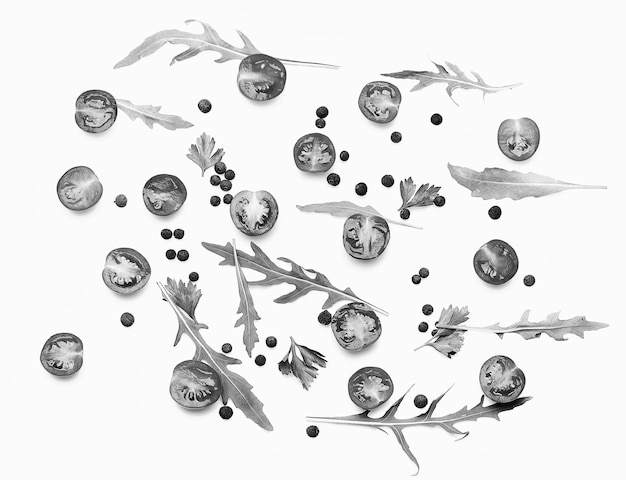In this black-and-white photo, a variety of food items are artfully arranged against a stark white background. At the forefront are sixteen cherry tomatoes, meticulously sliced in half, with their juicy interiors and seeds prominently displayed to capture the eye. These tomato halves are evenly dispersed throughout the composition. Interspersed among the tomatoes are approximately 10 to 15 arugula leaves, contributing to a sense of natural randomness with their varied placements—horizontally, vertically, and diagonally. Adding to the intricate visual texture are clusters of 20 to 40 small, dark spheres, possibly berries or seeds, scattered amid the tomatoes and leaves. The entire arrangement, presented in shades of gray and black, creates a striking and detailed still life against the contrasting white background.